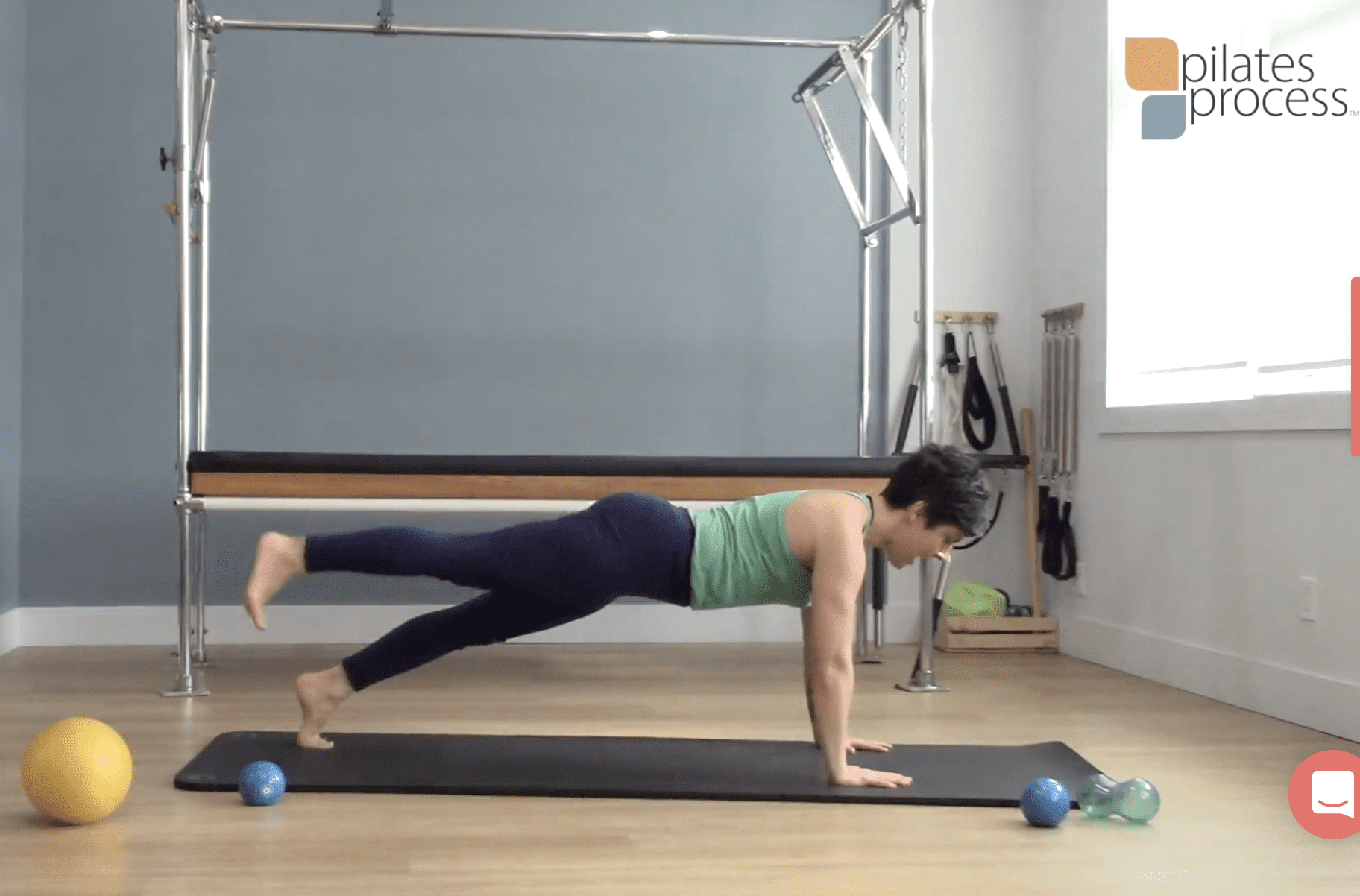A woman, appearing to be in her 30s or 40s, is pictured performing a floor exercise on a black yoga mat in a room that has the appearance of a private gym or physical therapy room. She is in a plank position, with her hands firmly pressed into the mat and her arms fully extended, her face angled downwards. Her left leg is extended back with the toes touching the mat while her right leg is raised straight into the air. The woman, who has light brown hair, is barefoot and wearing black leggings with a light green tank top. Surrounding her are several pieces of equipment, including three small balls near the top of the mat, a single smaller ball at the bottom, and a large yellow ball a bit farther away. Additional equipment such as a Pilates machine and resistance bands affixed to the gray wall are also visible. The room features light brown wooden flooring, gray walls with white trim, and a large window on the right side. Bright light streams through the window, which bears the inscription "Pilates Process." The atmospheric setting, the careful arrangement of equipment, and the woman's focused pose suggest a dedicated space for structured and intense workout routines.